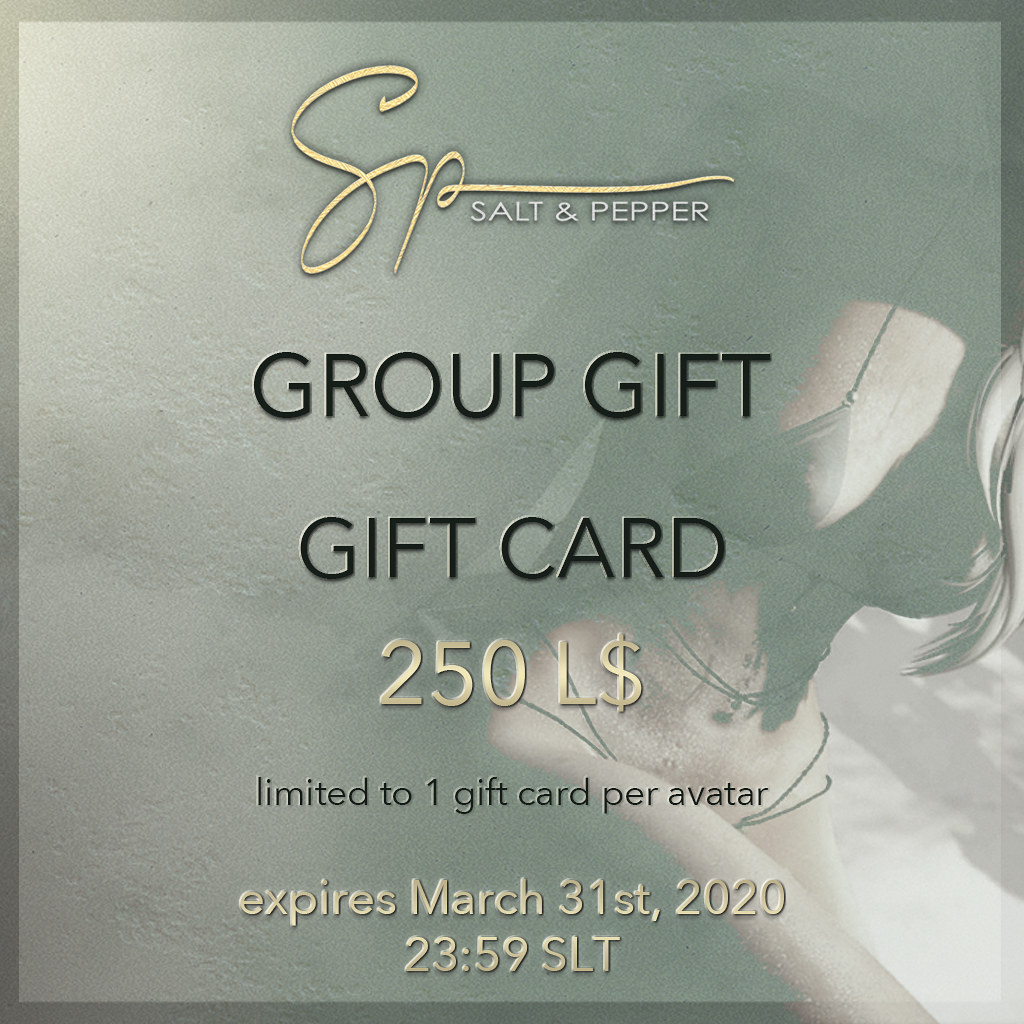The image features an advertisement for a group gift card valued at 250L for a spa called Salt-N-Pepa. The background is a cement grey wall adorned with a silhouetted woman in a brown, skimpy bikini; her long hair drapes over her body, obscuring her face. The text on the ad employs a mix of curvy gold and black fonts, stating "Salt-N-Pepa" followed by "Group Gift Card" in all capital letters. Further details specify the gift card's value of 250L, limit of one per avatar, and an expiration date of March 31st, 2020 at 23:59 SLT. The overall design is simple yet eye-catching.